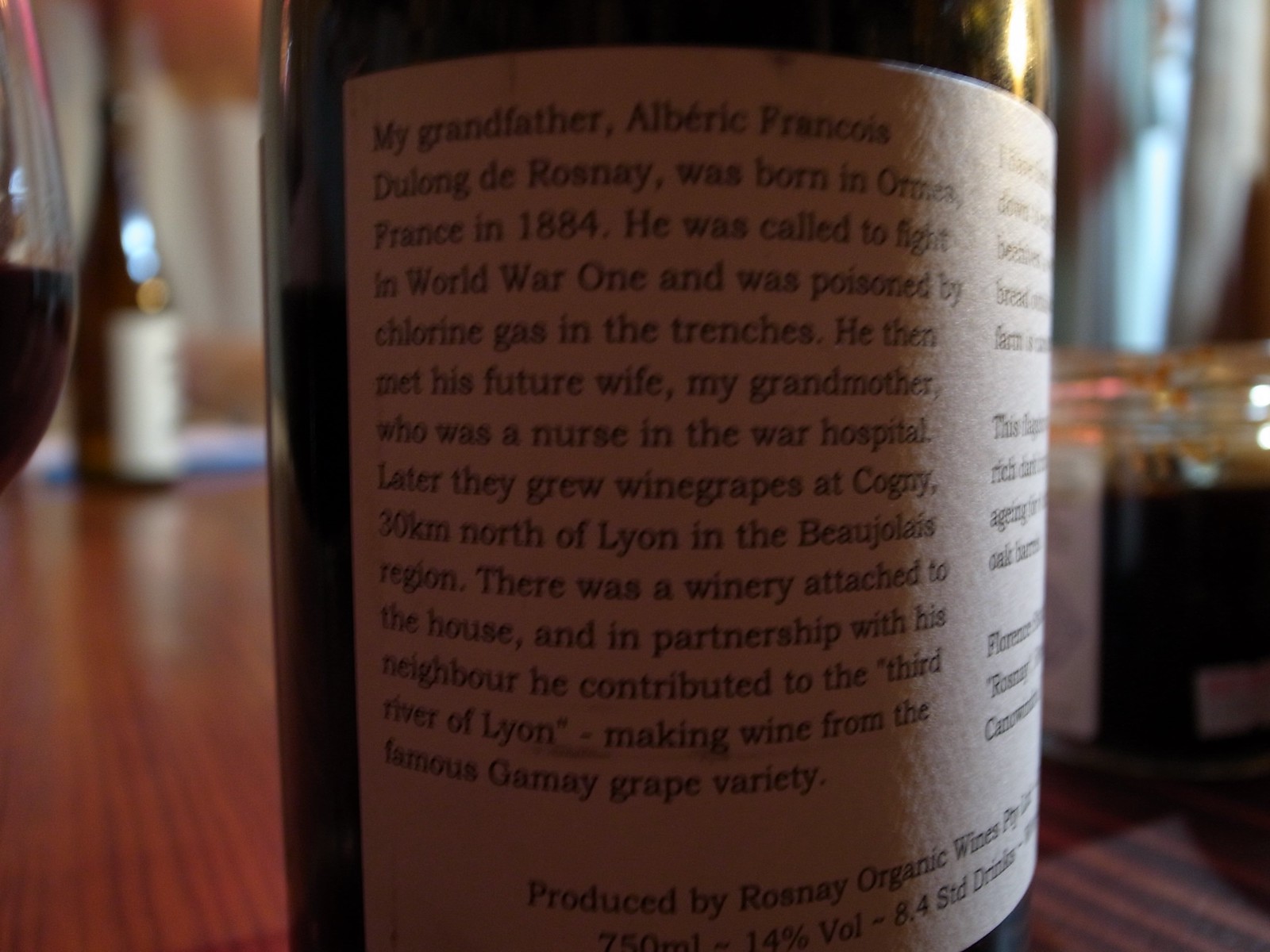This full-color indoor photograph captures a close-up of a wine bottle label that narrates the family history behind the bottle. The foreground of the image prominently displays the label with black print, while the background is out of focus, revealing a wooden table, a glass of wine to the left, and another wine bottle. An out-of-focus candle or similar item in a glass jar appears on the right. The label recounts that the grandfather, Alberic François Doulon de Rosnay, was born in Ornias, France, in 1884 and fought in World War I, where he was poisoned by chlorine gas. He met his future wife in a war hospital where she worked as a nurse. They later cultivated wine grapes in Cogny, 30 kilometers north of Lyon in the Beaujolais region, contributing to the Third River of Lyon wine production with their Gamay grape variety. The label also indicates that the wine is produced by Rosnay Organic Wines, and the bottle is 750 milliliters with an alcohol content of 14%, equating to approximately 8.4 standard drinks.